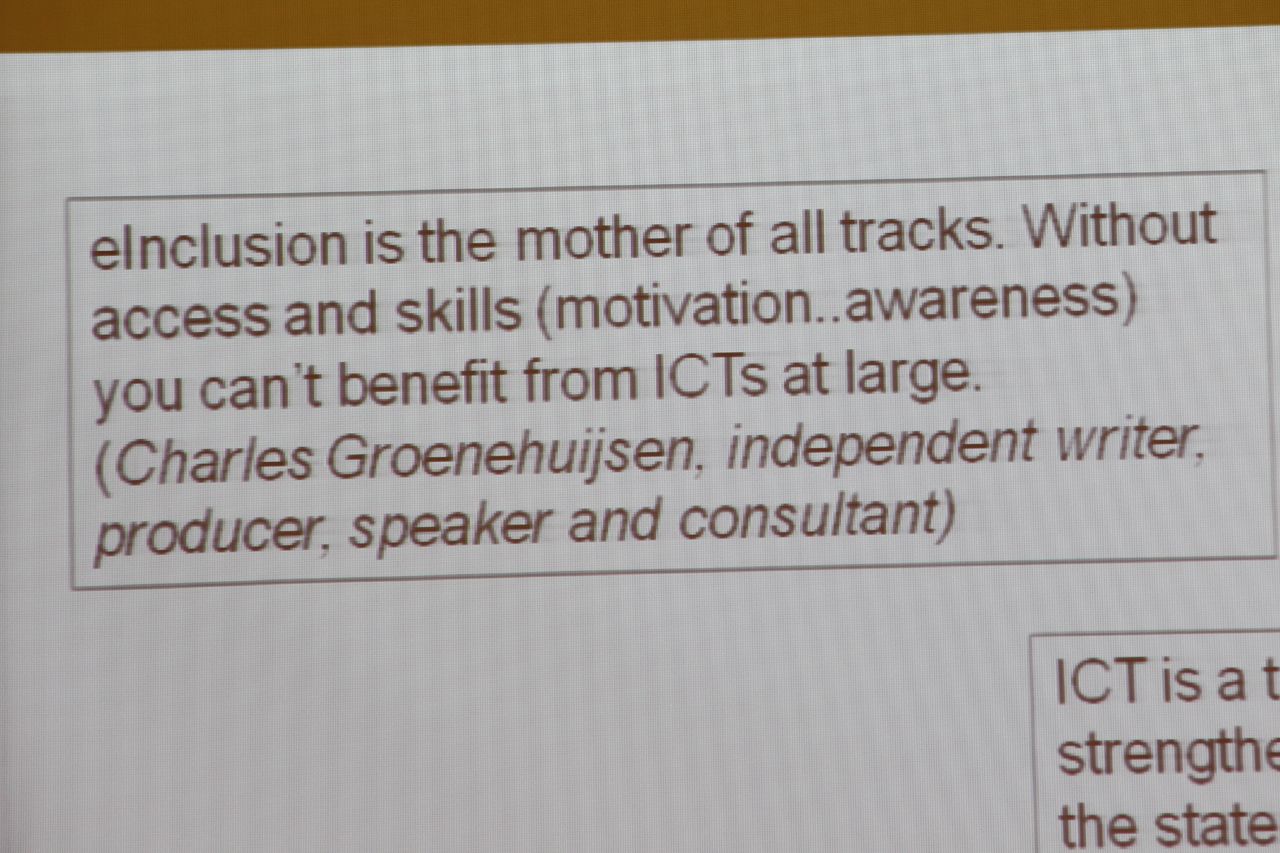The image depicts a digital screenshot of a web page or document featuring a white background with a brown header at the top. The content is partially cut off, but the visible text reads: "E-inclusion is the mother of all tracks. Without access and skills (motivation, awareness), you can't benefit from ICTs at large." The quotation is attributed to Charles Groenhuijsen, identified as an independent writer, producer, speaker, and consultant. The bottom right corner of the image shows the partial text, "ICT is a... strength... the state," suggesting further information about ICT is truncated. The screenshot exhibits digital noise typical when capturing a computer screen, with visible grid lines and feedback artifacts.